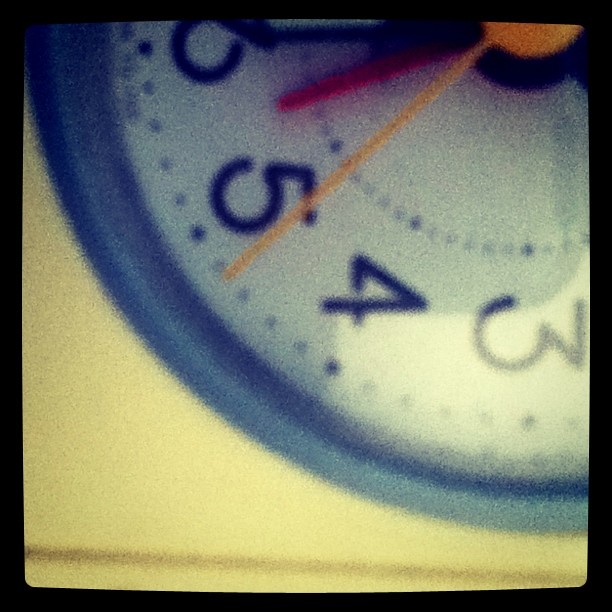This image is a grainy, fuzzy close-up photograph, likely cropped, capturing a quarter of a classic circular clock face from 3 to 6. The clock has a yellow background with tiny black dots, and its white clock face features numbers in black and gray shadow. The hands of the clock include a prominent yellow longhand just before the five, a shorter red hand slightly after the five, and a yellow ticking hand. The photograph includes a thin black border surrounding the image, giving it a vintage appearance against an off-white wall background.